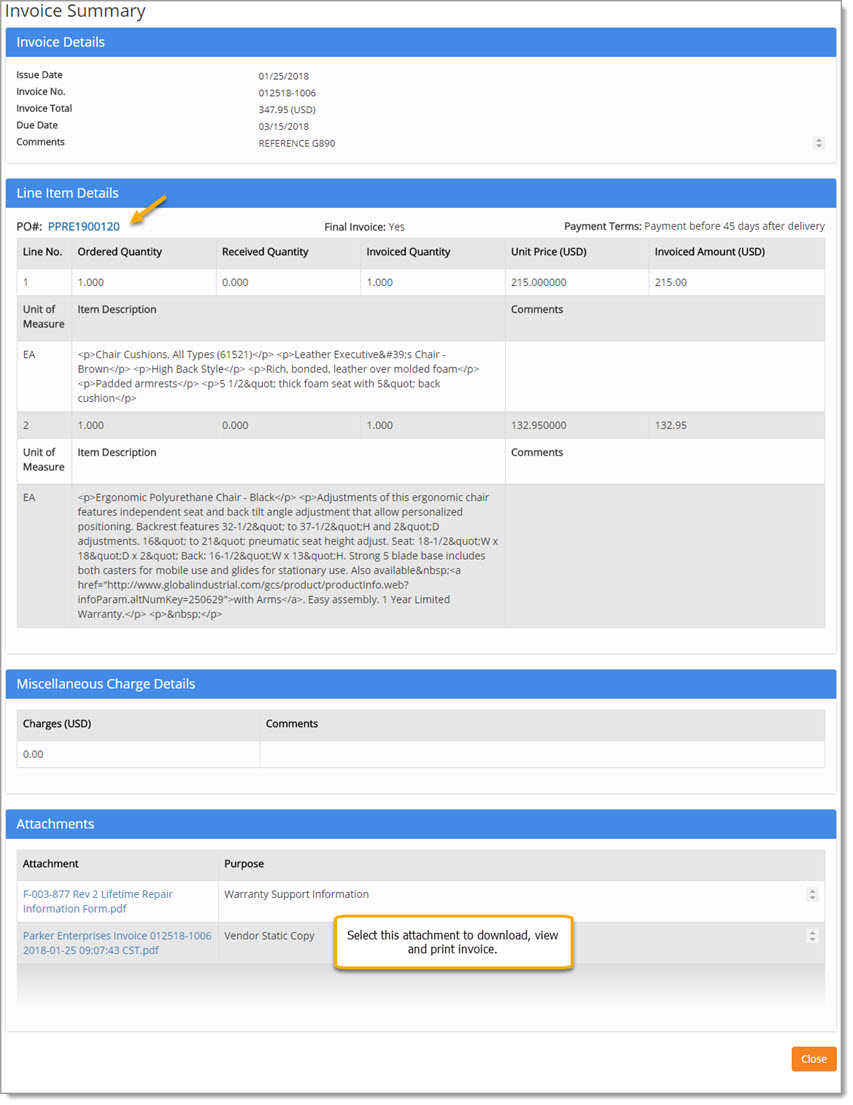The image depicts an invoice with a structured layout and a clear hierarchy of information. 

At the top left corner, there's a section labeled "Invoice Summary." Below it, within a blue-bordered area titled "Invoice Details," information is provided, including the invoice date, invoice number, invoice total, due date, and comments. 

Further down, another blue-bordered section labeled "Line Item Details" presents the Purchase Order (PO) number, highlighted by a yellow arrow. The PO number is PPRE1900120. This section also includes columns for line number, ordered quantity, received quantity, invoice quantity, unit price, invoice amount, unit measure, and item description.

Following this, there is a "Miscellaneous Charge Details" section, also bordered in blue, indicating there are no additional charges.

At the bottom, a blue-bordered "Attachments" section outlines available attachments and their purposes. There is a highlighted area in yellow in the middle of this section, instructing to "Select this attachment to download, view, and print invoice." This appears to correspond to the earlier mentioned yellow-highlighted PO number. Finally, an orange "Close" button is located at the bottom right corner of the layout.

This detailed and organized layout ensures that all necessary invoice information is clear and accessible.